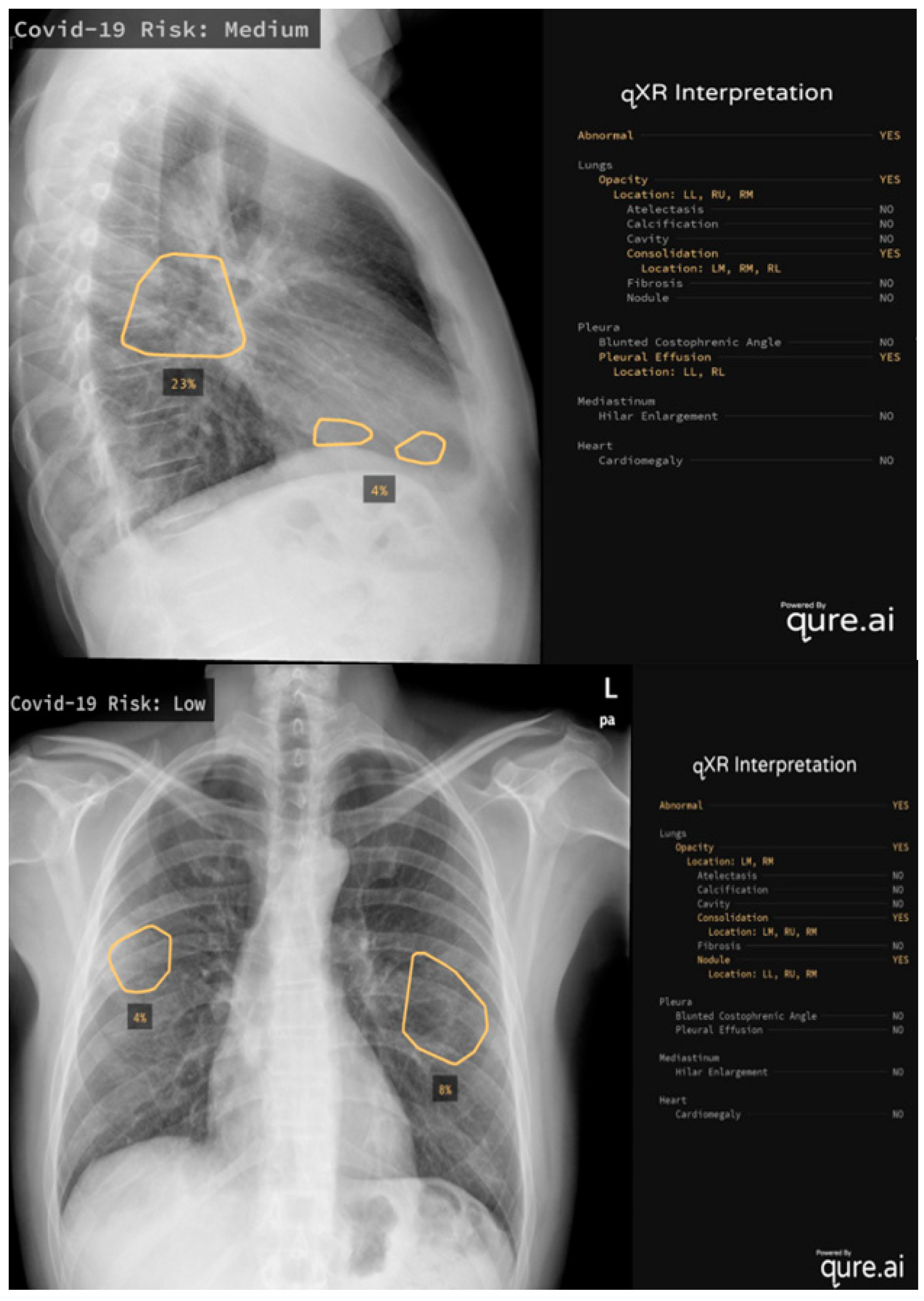This image features two stacked medical scans, each illustrating different views and risk assessments related to COVID-19. The top portion of the image is a side view torso scan, presenting a primarily black background with the title "QXR Interpretation" in white text at the top. This scan is a blurry, white x-ray marked by three orange circled areas, labeled with percentages, indicating key points of interest. Text in the upper left corner declares a "COVID-19 Risk Medium" assessment.

Beneath this, the lower portion of the image displays a frontal chest x-ray, clearly outlining the ribs and shoulders. In this scan, two orange circles, also labeled with percentages, highlight significant areas. The upper left text here denotes a "COVID-19 Risk Low." Both images feature detailed annotations on the side, seemingly powered by an AI platform, Qure.ai, to aid in analyzing the risk and identifying abnormalities within the scans.